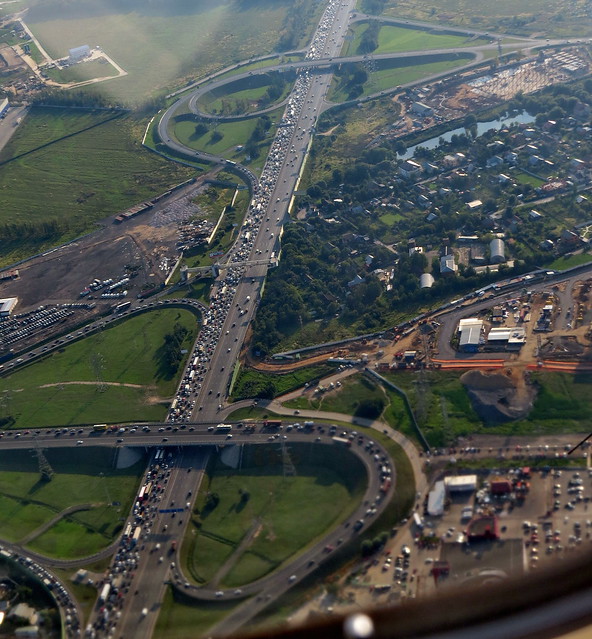This is a crisp and clear aerial photograph taken from a helicopter window, as evidenced by the visible silver trim at the bottom edge of the image. The vantage point provides a sweeping view of a bustling urban area below, highlighting several interstates adorned with numerous vehicles, including darker and lighter-colored cars, as well as a couple of buses navigating an overpass. The landscape features a mix of industrial zones and residential areas, identifiable by the tops of various buildings in burgundy, orange, and white hues. Verdant green trees and patches of grass intersperse the concrete jungle, adding a natural element to the scene. The photograph's sharpness reveals even minute details, such as dirt spots on the reflective surface of the helicopter's window, contributing to the authenticity of capturing a vivid urban tapestry from above.